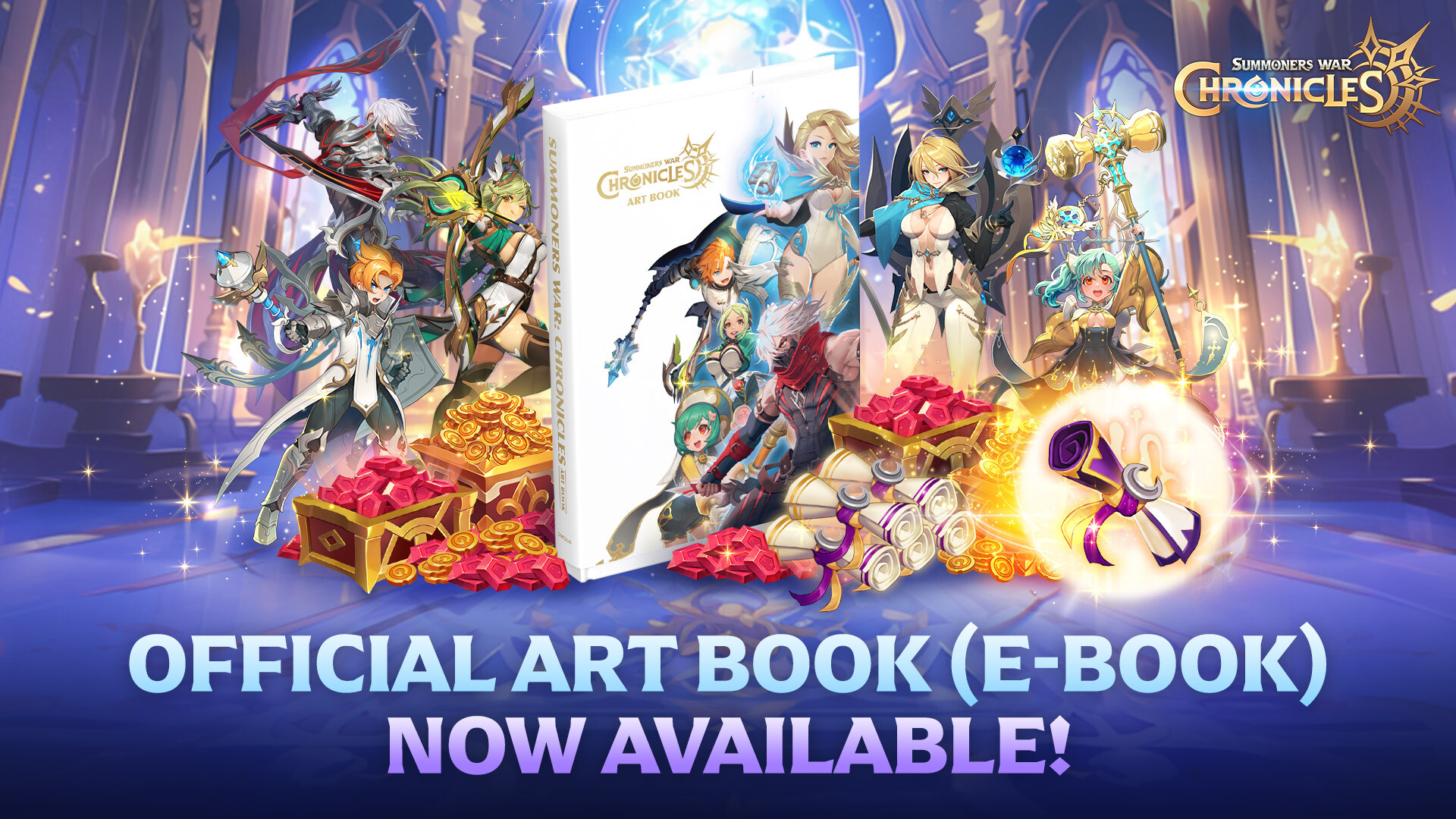This graphic advertisement depicts an anime-style image promoting the "Summoners War Chronicles" Official Art Book (E-Book). The focal point is a white compilation book centered in the image, featuring illustrations of various manga-style characters, some of whom are also positioned around the book. These characters, consisting mainly of fairy-like women with pointed ears and ornate weapons like maces and arrows, are set against a high-contrast, blue and gray fantasy backdrop that appears to be inside an illuminated castle.

To the left of the book, there are treasure chests brimming with red gems and gold coins, adding to the fantasy theme. The top right corner of the image displays the "Summoners War Chronicles" logo, while at the bottom, bold blue text announces, "Official Art Book (E-Book)," followed by a purple declaration, "Now Available." This advertisement effectively combines vivid, cartoonish aesthetics and intricate fantasy elements to draw attention to the newly available art book.